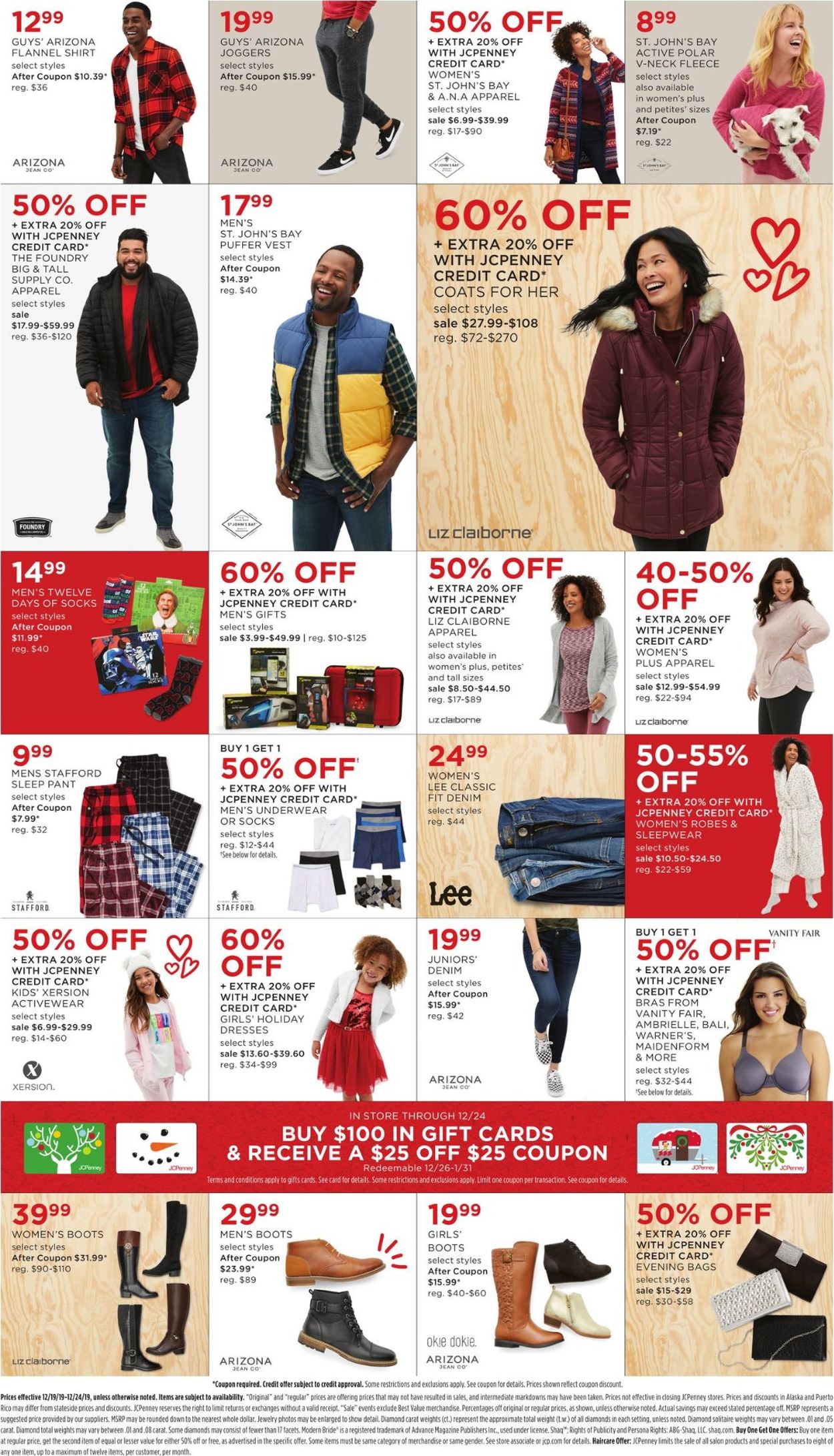This is a detailed and cleaned-up description of the digital advertisement screenshot:

The screenshot is of a digital advertisement for JC Penney, primarily featuring a red, white, and gray color scheme. The ad is segmented into a 4x6 grid, with a total of 24 squares, each displaying various promotions and images. 

- The first square features the promotion "$12.99" for a men's Arizona flannel. The image accompanying this promotion shows an African American male wearing an open black and red flannel shirt. 
- The second square displays a price of "$19.99" in red numbers, indicating a men's Arizona item, likely featuring a pair of skinny jeans.
- The third square in the grid is a white box with text in red that reads "50% off," and an additional offer of an extra 20% off when using a JC Penney credit card. This promotion applies to women's St. John's Bay and A&A apparel. The image shows a woman on her cell phone wearing a flannel shirt and a coat.

Each square in the advertisement focuses on either a price point or a discount offer, with clear images of the clothing items featured.